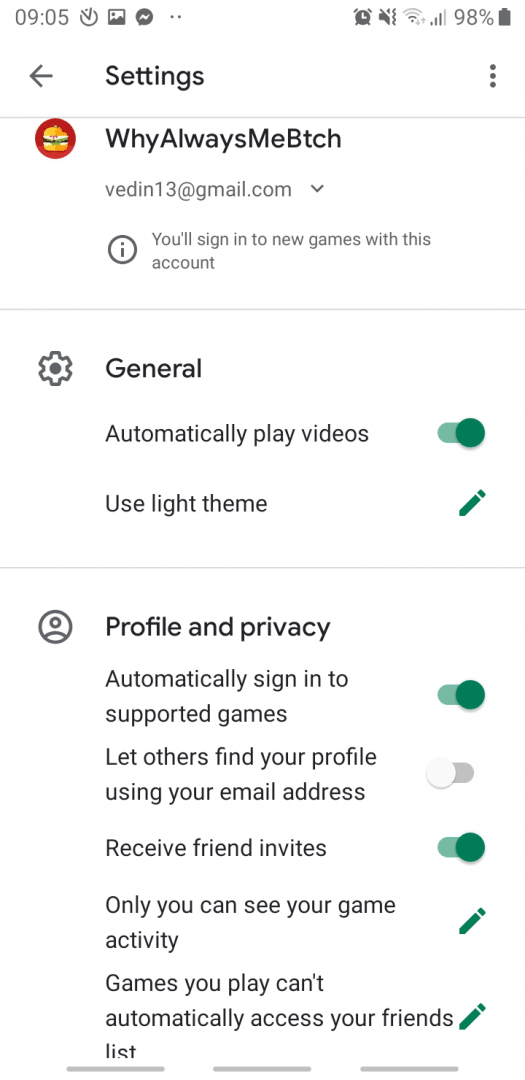In the screenshot of a mobile phone displaying game settings that resemble Google settings, the time reads 9:05 AM. A clock icon is noticeable next to the timestamp. Alongside it, various icons are visible, including one for pictures, a chat icon, two dots, and an alarm signifying that an alarm is set. Additional icons indicate that the sound is muted, the device is connected to Wi-Fi with full signal strength (four bars), and the battery is at 98% charge. 

In the header, there is a left arrow symbol directing backward, labeled "Settings." On the right side of the header, there are three vertically aligned dots, possibly indicating a menu or additional options. A gray line separates this section from the next, which contains a round circle icon with an image resembling a hamburger, accompanied by the phrase "Why Always Me BTCH" (with "BTCH" presumably an abbreviation for a censored version of "bitch").

An email address, VDNVEDIn13@gmail.com, is displayed with a drop-down arrow beside it. An information icon (a lowercase "i" inside a circle) is present, alongside the message, "You'll sign in to new games with this account."

A separating line introduces the next category labeled "General," accompanied by a gear icon. Within this section, the option to "Automatically play videos" is toggled on. There's also an option to "Use light theme," which has a pencil icon next to it, indicating that it can be edited.

Further down, another light gray line separates the "Profile and Privacy" section. Here, there's an icon of a person inside a circle. Options within this section include "Automatically sign in to supported games," toggled on, and "Let others find your profile using your email address," which is toggled off. The setting to "Receive friend invites" is toggled on, and it states that only the user can see their game activity, with a pencil icon next to this option. It also notes that games cannot automatically access the user's friends list, which again comes with an adjacent pencil icon for editing. Three gray lines conclude this section.